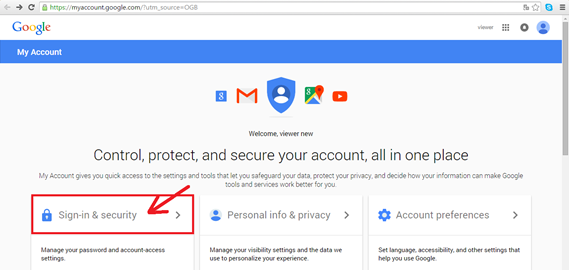A screenshot from the Google Account management webpage displaying a user's account page. The header text reads, "Welcome, you are new. Control, protect, and secure your account all in one place." Three main menu options are prominently featured: "Sign-in & Security," "Personal Information & Privacy," and "Account Preferences." The "Sign-in & Security" tab is highlighted with a red box, and a red arrow points directly to it, indicating that it is the focal action area. This visual marker suggests an instructional purpose, guiding users on how to manage their password and account access settings as part of an informative step-by-step process.